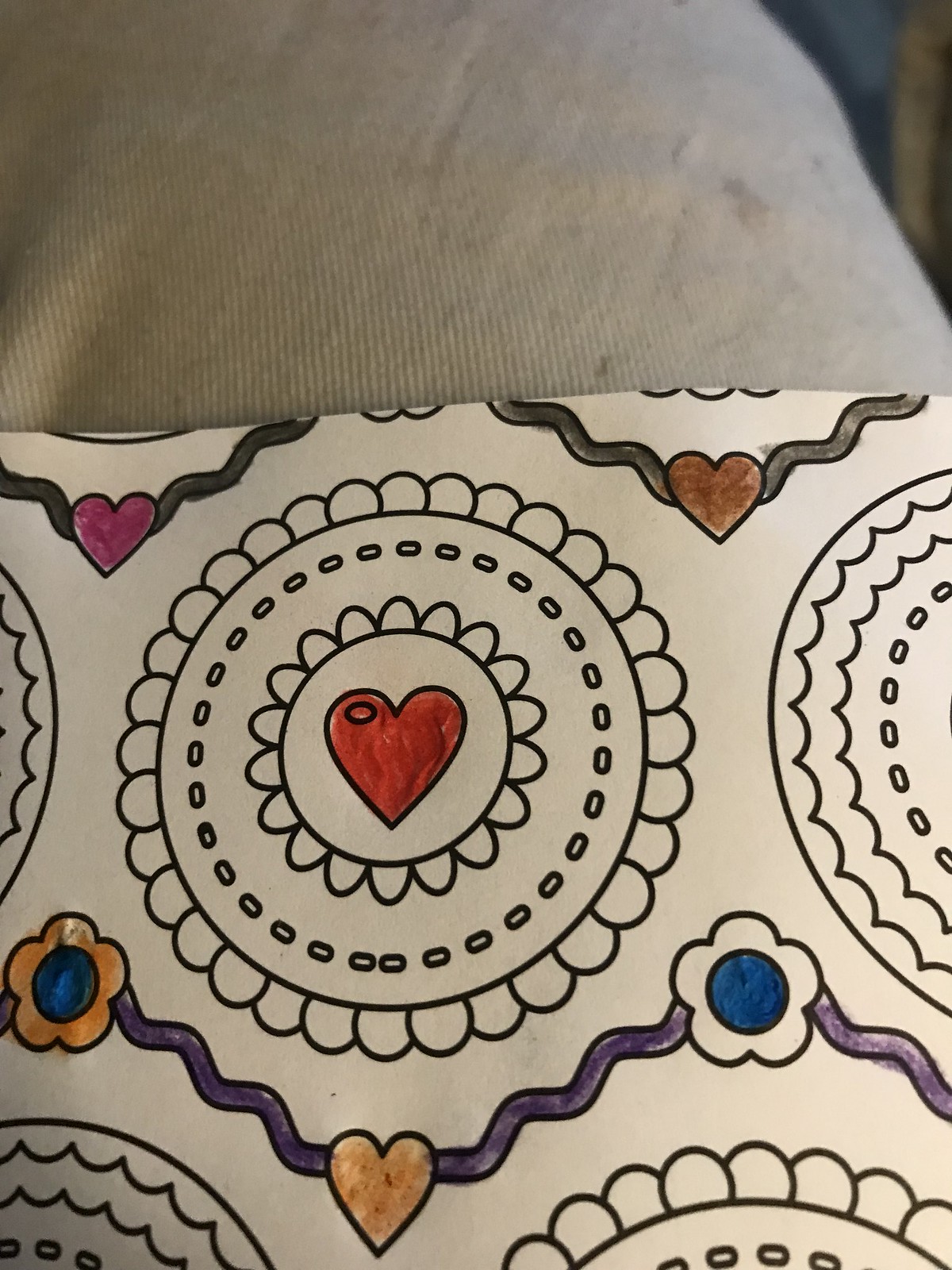This photograph captures a section of a coloring page featuring intricate patterns and designs. The upper half of the image displays a white background, reminiscent of a corduroy fabric with very thin lines, contributing a textured appearance. The upper right-hand corner introduces contrast with a black area intersected by a brown line running vertically.

Dominating the lower three-quarters of the photograph is a detailed series of patterns centered around a vividly colored red heart. This heart is prominently outlined in black and filled in with a vibrant red hue. Encircling the heart is a series of small half-circles, adding a decorative border. Further out, a ring of outlined ovals forms another concentric circle, which is also bordered by a single black line. Surrounding the outer edge of this black line is an additional series of half-circles.

The pattern repeats horizontally across the page, interspersed with smaller motifs. Between the rows of central designs are alternating small hearts and daisy-like flowers, interconnected by wavy lines. The interconnecting line at the top is colored green, while a pink heart adorns the left side and a brown heart the right. At the bottom, a yellow daisy with a blue center stands out, connected by a gray line to a brown heart, which in turn links to another daisy with a blue center, continuing the detailed and colorful theme of the page.